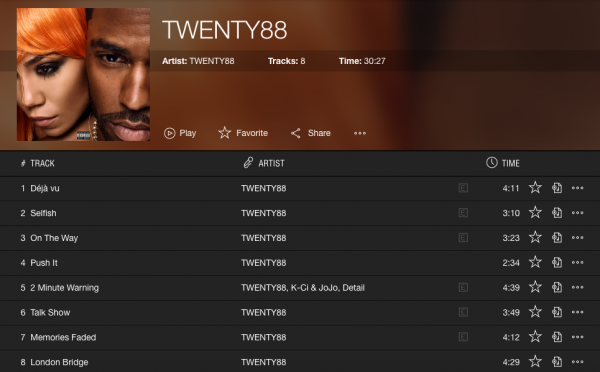The image showcases a close-up of two individuals featured prominently on a music website, positioned in the upper left-hand side. The individuals are a male on the right and a female on the left, both captured in a side-by-side format with portions of their faces cut off—specifically, the left side of the male's face and the right side of the female's face. The image emphasizes their expressions, creating an engaging focal point. 

To the right of their faces, the name "2088" appears, likely indicating the artist's name, accompanied by details of their work: "8 tracks" with a total playtime of "30 minutes and 27 seconds." Below this summary, a list of the eight tracks is visible, each entry displaying the respective track's name, the artist (presumably 2088), and the duration of each track.